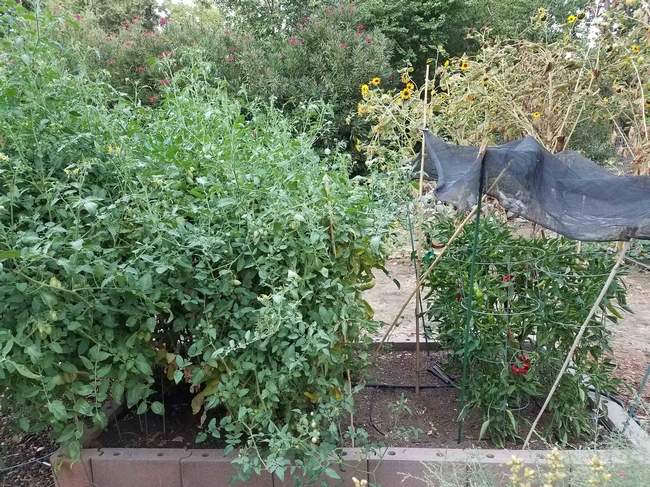In this image, we observe a serene, lush forestry area that captures the essence of a well-maintained garden. At the very bottom, there is a neat arrangement of interlocking grayish bricks. These interlocking stones have distinct lips that connect each piece, and one full-size brick prominently features two perforations—one on the left and one on the right. 

As the scene extends from left to right, it reveals a raised garden bed encircled by these interlock stones. The bed itself is filled with rich, brown soil and is dotted with several sticks protruding from the earth. Centrally positioned within this garden bed is a round, metal plant support cage, typically used for tomato plants to prevent them from toppling over. This support structure is secured by a gray metal rod, ensuring the cages remain upright.

Covering the area, there is a delicate gray mesh for additional plant protection. On the left side of the garden bed, a dense cluster of green bushes creates a vibrant contrast to the earthy tones of the soil and stones. In the backdrop, an array of tall, green forest trees stretches out, enhancing the lush greenery of the scene. Central to the garden bed, several blooming flowers with yellow petals and black centers add a splash of bright color to this picturesque forestry area.